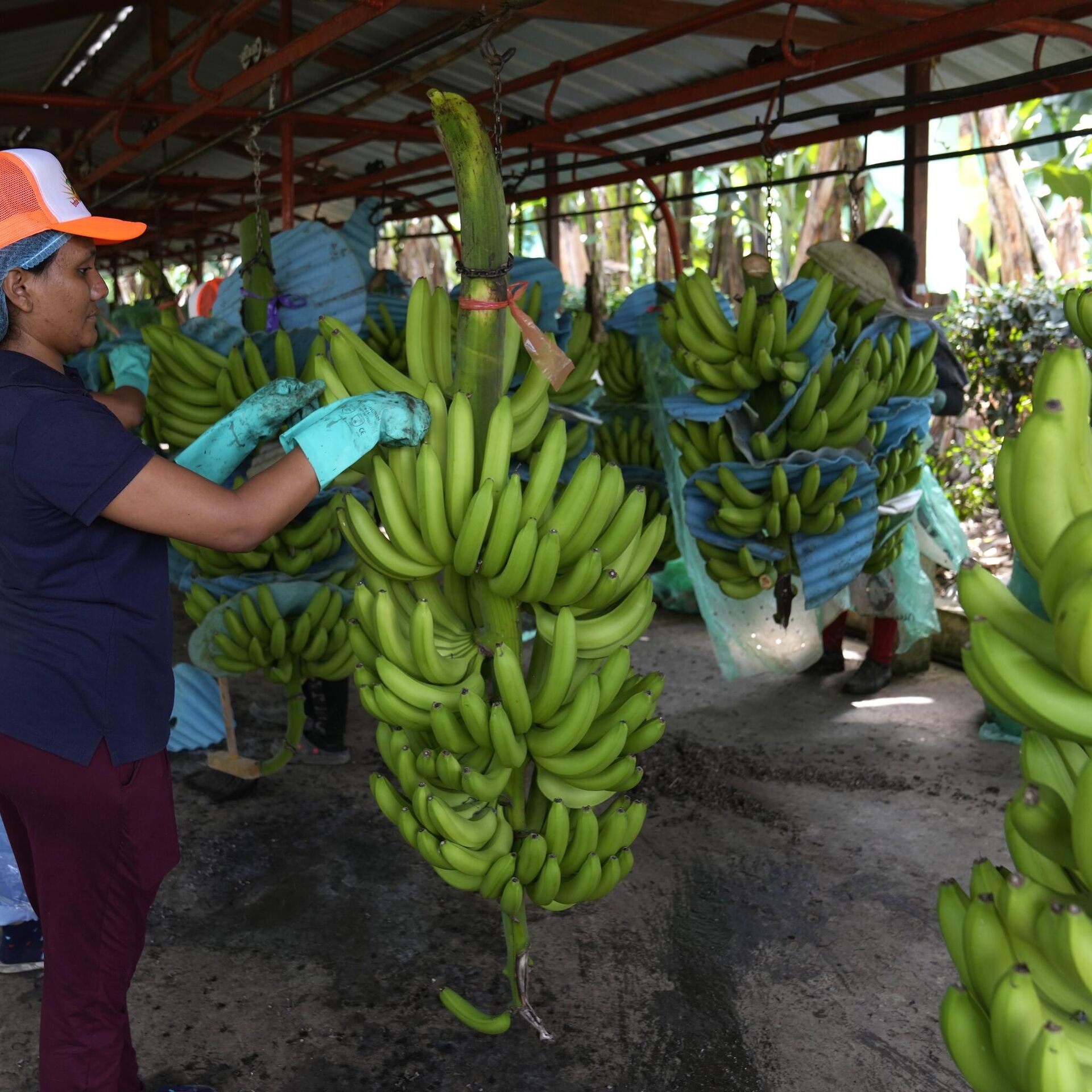This outdoor image is of a tropical banana collection center with an open-air setting, featuring a tin roof supported by black and brown rafters. Large bunches of green bananas hang from the roof on chains, still attached to their stems. Two workers are present, busily handling the bananas. The first worker, positioned to the left, is a dark-complexioned woman wearing a bright orange baseball cap with a white front, a navy t-shirt, red pants, and mid-arm-length rubber gloves. She appears to be arranging the bananas. In the background, another person is partially visible, wearing a skirt and seemingly using blue tarp sections to wrap and separate the banana bunches. The tropical ambiance is underscored by foliage in the distance and the lightweight clothing of the workers. The ground appears to be dirt, further emphasizing the rustic and natural environment of this banana farm. Rows of bananas hanging in the air showcase the abundance of the harvest.